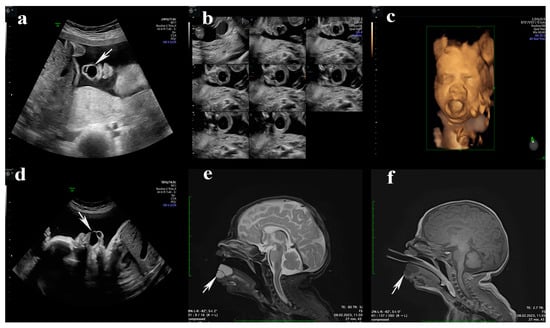This image is a detailed composite of six different scans of a fetus labeled A through F, arranged in a grid with three at the top and three at the bottom. 

- Image A is a black-and-white ultrasound showing a trapezoidal view of the fetus, with light gray blotches in the center and an arrow pointing to a specific area, possibly the head or umbilical cord.
- Image B displays a collection of eight smaller ultrasound images, zooming in on specific parts of the fetus, arranged in rows.
- Image C features a 3D scan in a brownish-yellow color, depicting a close-up of the baby's face with its mouth open, eyes visible, and part of its ears.
- Image D presents another black-and-white ultrasound from a different angle, showcasing the side profile of the baby, possibly lying on its back.
- Image E appears to be an x-ray of the fetus's head in profile, revealing internal structures such as the brain and brainstem.
- Image F, similar to E, shows an x-ray of the baby’s head and neck area, this time highlighting the external structure with something extending into the mouth, possibly a medical instrument.

All images are highly technical, primarily in shades of black, white, and gray, except for the 3D scan in C which adds a brownish tone. They collectively provide a comprehensive overview of the fetus from multiple perspectives and stages of scanning technology.